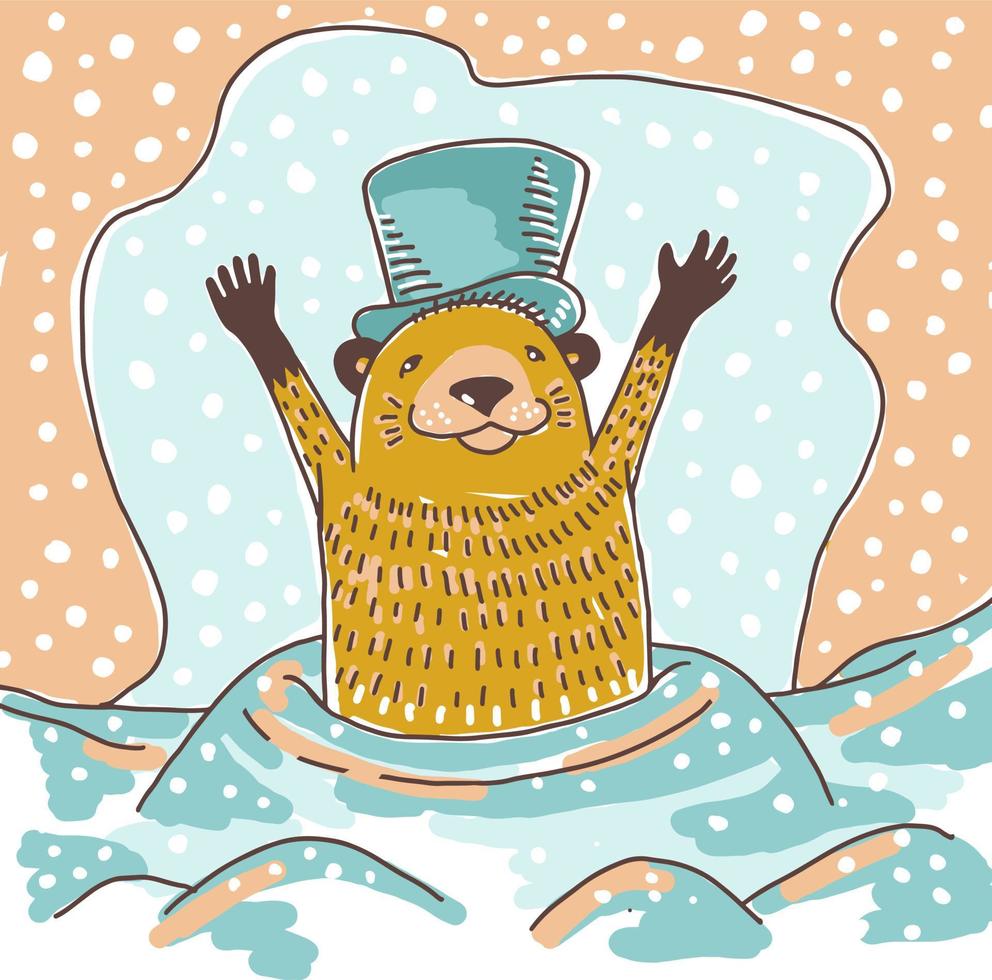This is an adorable digital artwork of a cartoon groundhog emerging from a hole in the ground. The groundhog, with its arms raised in the air, sports a dark blue or turquoise top hat and has a fur-like texture indicated by fine lines. Its fur is a mix of darker brown on the arms and a lighter brown overall. The groundhog is surrounded by a whimsical winter scene with snow represented as falling white dots against a light blue and pinkish sky. The ground itself is a vibrant blend of dark turquoise, light turquoise, and brown, with snow covering the area around the hole, adding to the wintery feel of the scene.